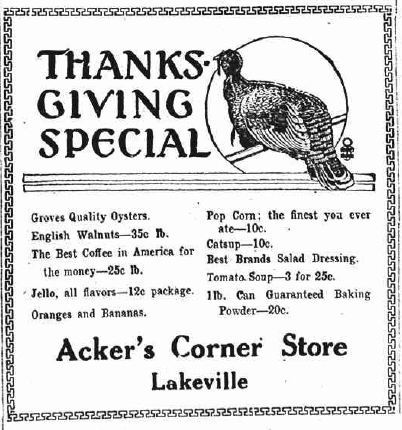This is a detailed black-and-white ad for Acker's Corner Store in Lakeville, showcasing a vintage Thanksgiving special. The design features an old-fashioned sign with intricate, chain-like detailing along the top and bottom edges of the rectangle. At the top left, "Thanksgiving Special" is written in a decorative font, accompanied by an illustration of a turkey roosting on a branch within a circle that frames most of its body, except the tail and a bit of the beak. Beneath the turkey are two slender parallel bars.

The menu is divided into two columns. The left column lists:
- Groves Quality Oysters
- English Walnuts, 35¢ per pound
- The Best Coffee in America for the Money, 25¢ per pound
- Jell-O, All Flavors, 12¢ per package
- Oranges and Bananas

The right column includes:
- Popcorn, The Finest You Ever Ate, 10¢
- Catsup (spelled the old-fashioned way with a "C"), 10¢
- Best Brands Salad Dressing
- Tomato Soup, 3 for 25¢
- One Pound Can Guaranteed Baking Powder, 20¢

At the very bottom of the sign, "Acker's Corner Store" is neatly detailed, with "Lakeville" centered beneath it. Judging by the listed prices and the overall design, this advertisement dates back to a bygone era, evoking a sense of nostalgia for a village store probably long gone by now.